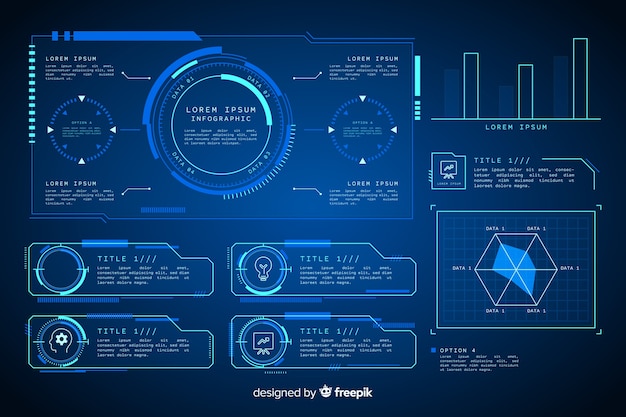This image showcases a detailed infographic blueprint with a dark blue background adorned with various graphical elements in different shades of blue and light green. At the top left, a prominent circular element displays the title "Lorem Ipsum Infographic" in the center. Surrounding this main circle are four smaller ones at the cardinal points (12, 3, 6, and 9 o'clock positions), each marked with white arrows. 

Below this primary section and extending to the right, there are multiple compartments of information. Directly beneath the main circle is a trio of squarish graphs of varying heights, rendered in light green. Adjacent to these graphs, a light green hexagonal infographic appears, adding a geometric variation to the design.

To the left, the blueprint contains a series of four circled icons, each containing distinct imagery: a blank circle, a circle with a light bulb, a circle with a person's face and a star, and a circle with a TV-like screen on a leg stand. Each of these icons is labeled "Title 1," indicating placeholders for customizable content.

At the very bottom of the infographic, the caption "Designed by Freepik" is accompanied by a small illustration of a face with pointed ears, eyes, and a mouth. Overall, the image represents a template-like infographic with sections explicitly designed for customization, making it a versatile guide for creating structured visual data presentations.